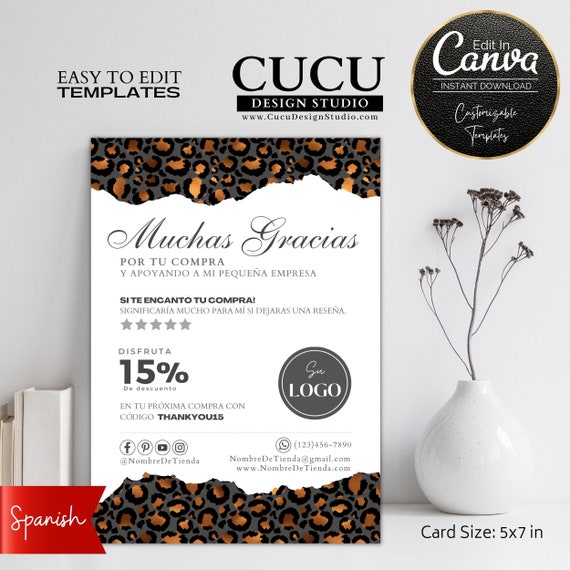This visually engaging advertisement showcases a sample template for designer cards, specifically measuring 5x7 inches. The cards prominently feature Spanish text, highlighted by a distinct small red ribbon in the bottom left corner labeled "Spanish." The top of the image bears the slogan "Easy to edit templates" followed by the branding details: "C-U-C-U. Design Studio" and the URL "C-U-C-U.DesignStudio.com." Additionally, it mentions the ease of editing in "Cavana" and the option for "Instant download."

Central to the image is an exemplary card, displaying Spanish writing and adorned with a stylish cheetah-patterned border on both the top and the bottom. To the right of the card, there is a minimalistic white base featuring a slender plant, adding a touch of natural elegance to the overall design.